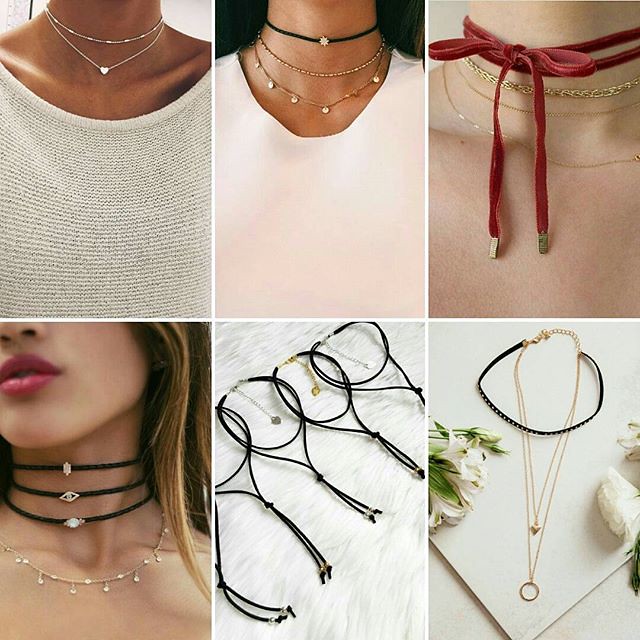The image is a detailed collage of six smaller rectangular photos showcasing various choker and necklace styles. The top-left shows the neck of a darker-skinned woman wearing a beige knit top, with two layered gold chokers, one of which features a small gemstone heart. Next to her, another darker-skinned woman in a light pink or salmon-colored top dons three small necklaces: a black band with a star-shaped gem, a simple gold choker, and a gold necklace adorned with tiny gems. The third image in the top row features a light-skinned woman sporting a unique combination of four pieces: a large red velvet choker tied in a bow with gold-tipped tassels, accompanied by three gold necklaces.

In the bottom-left, an Asian woman with shoulder-length brown hair and red lipstick wears four neck adornments: three black chokers each featuring a small gem or motif in the center, and a separate short gold necklace adorned with dangling stones. The fifth image displays a collection of black choker necklaces laid out on a plain white background, resembling lacy or lanyard-like materials. The final photo presents a black choker and two longer gold necklaces with distinct pendants—a hoop and a heart—arranged on a white background with delicate floral accents on either side. Each image highlights the intricate design and variety of the chokers, emphasizing their elegant and fashionable appeal.